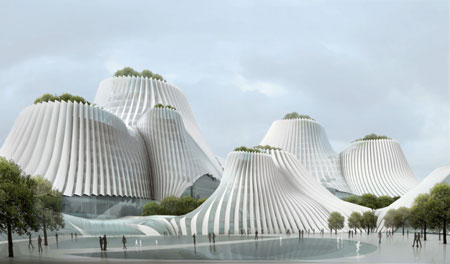The image is a 3D color architectural rendering of the Taichung Convention Center featuring six white, conical dome structures resembling volcanoes with distinct fluted, vertical ridges creating a pleated pattern on their surfaces. The structures are arranged with three on the left, two wider ones centrally placed towards the bottom, and two taller ones in the back on the right. Each dome has a flat top adorned with patches of lush green garden areas. In the immediate foreground lies an ice skating rink that spans the width of the image, its ice appearing solid but partially melting in the center. A visible frozen path runs through the center of the rink, where people can be seen walking or skating. The scene is framed by smaller trees on both the left and the right, with a clear, blue sky providing a crisp, clean backdrop. The whole setting exudes a serene, well-maintained atmosphere, capturing both natural and architectural beauty.